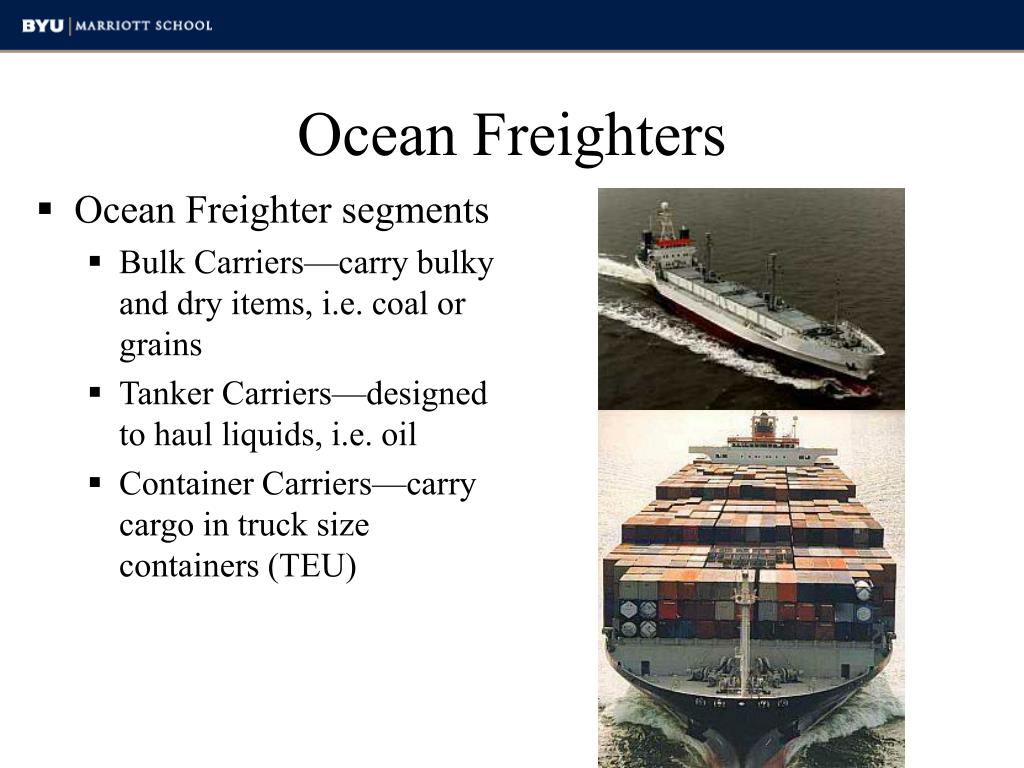The image resembles a PowerPoint slide primarily displaying information about ocean freight liners from the BYU Marriott School. The topmost section features a horizontal dark navy strip with the text "BYU Marriott School" in white, prominently on the left side. Centrally positioned below this strip, the title reads "Ocean Freighters" in black text. On the left-hand side, detailed bullet points discuss various ocean freighter segments: Bulk Carriers that transport bulky dry items like coal or grains, Tanker Carriers designed to carry liquids such as oil, and Container Carriers that haul truck-sized containers (TEUs). The right-hand side of the slide showcases two images of ships. The upper image displays a ship on the water with one level of storage containers and a white control station at the back. The lower image provides a closer view of another ship cruising through the water, loaded with containers stacked three to four levels high, covering the entire deck.